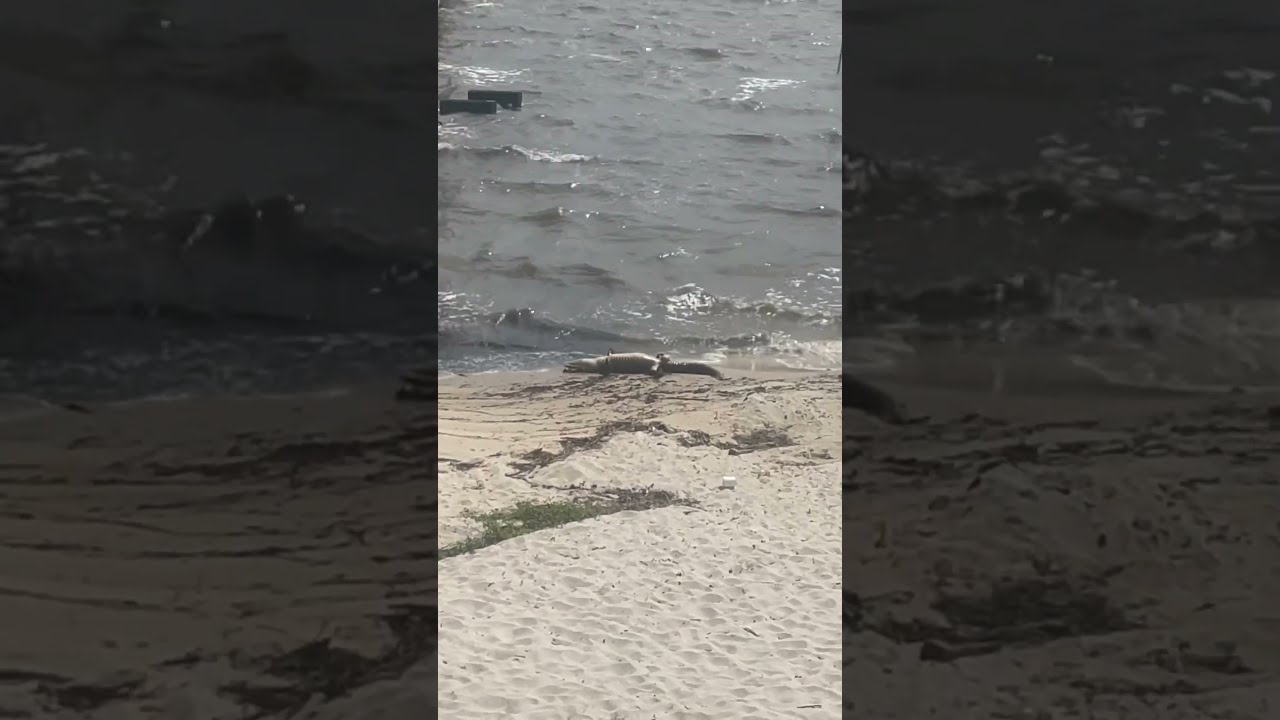The image is a postcard-style composition segmented into three parts with differing levels of brightness. The central panel, which is brighter and more detailed, displays a beach scene with beige sand occupying the lower half, interspersed with green vegetation and some debris, possibly a sea creature, washed up on the shore. The sand transitions into water where a seagull can be seen flying at a slight angle, its wings fully outspread. There is a poignant element to the scene due to what appears to be a dead alligator or sea creature lying on its back on the sand with its mouth open, adding a somber tone. In the distance, darker rectangular objects, perhaps debris or remnant beams, float in the water near the horizon. The left and right panels of the postcard are dimmed and zoomed-in sections of the central image, highlighting the waves and water with less detail than the central part, giving an overall fragmented and melancholic atmosphere to the scene.